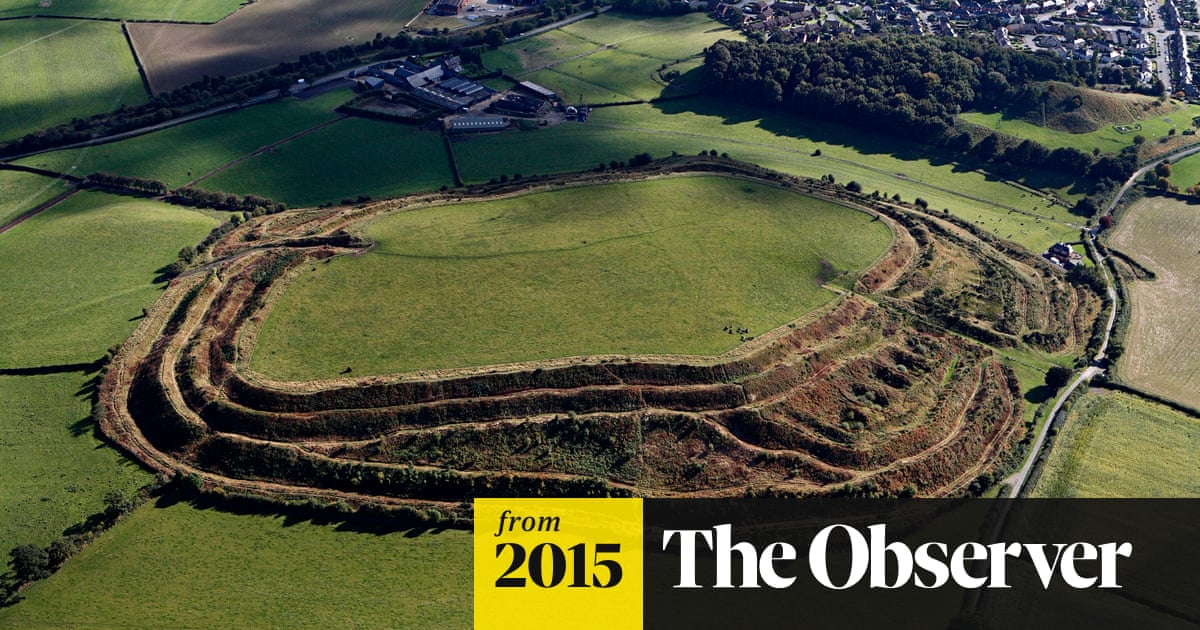This aerial shot, likely taken around 2015 and possibly featured in an article from "The Observer," captures a unique landscape from high above. Dominating the scene is a raised, green, grassy area situated in the center of the frame, which appears to be a hill or a plateau. Surrounding this elevated patch are several layers of descending trails or ridges, giving the impression of terracing, which could be indicative of a mining operation, an archaeological dig, or some other kind of land modification.

On either side of this raised central area, trails or paths extend through the grass, leading up and down the hill. The landscape surrounding the central hill is divided into various sections, accented by rows of trees that delineate different fields or properties.

In the background, the upper left corner features some buildings, possibly part of a residential or industrial complex, while the top right corner shows machinery and hints at a nearby neighborhood with a grid-like street pattern. Visible on the bottom left of the photo are two overlaid boxes: a yellow one inscribed with "from 2015" and a black one labeled "The Observer" in white text. This detailed and layered image offers a comprehensive view of an intriguing raised landform amidst a diversified terrain.